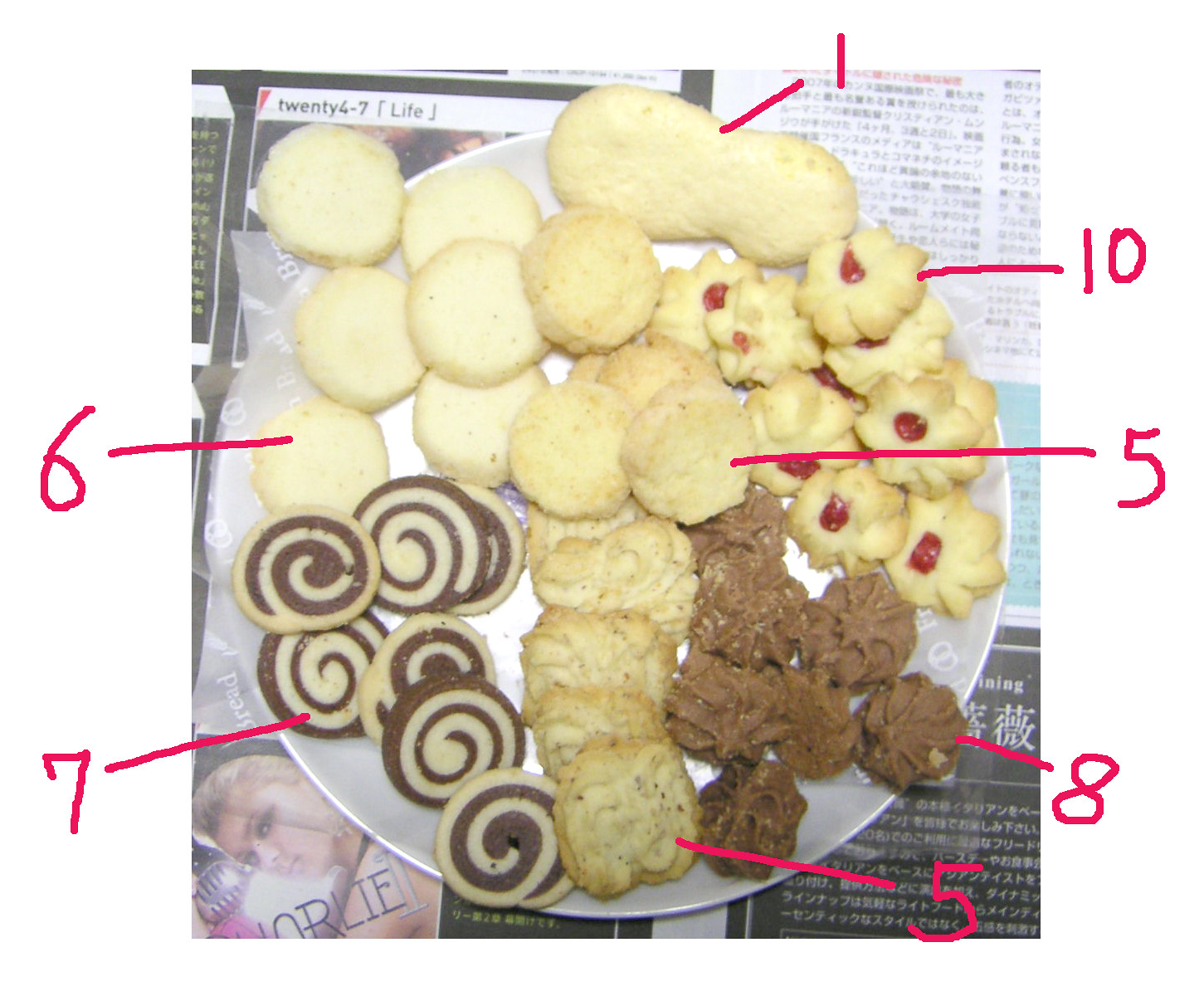This image depicts a round white plate filled with a variety of intricately designed cookies, each labeled with numbers. The plate is set on a paper background with Asian writing, suggesting an Asian influence or locale, such as a small cafe. The cookies, presumably from different assortments, feature unique shapes and colors. The number one cookie appears to be a large, cream-colored sugar cookie. Number five shows up twice – one is a small brownish-tan butter cookie while the other has black dots. Number six is a plain circular vanilla cookie. Number seven is a striking chocolate and vanilla swirl cookie. Cookie labeled eight is a round chocolate cookie with scalloped edges. Number ten is a shortbread cookie with scalloped edges, possibly adorned with a raspberry topping. Each cookie stands out with its distinct look, enhancing the overall visual appeal.